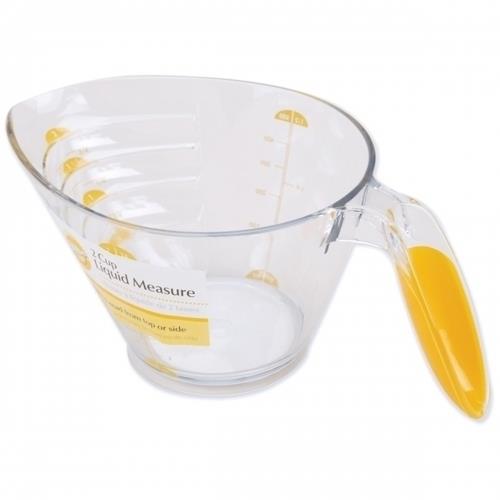This is a detailed image of a liquid measuring cup made from clear plastic with a white background, giving it a floating appearance typical of product photos on e-commerce sites. The cup has a yellow decoration in the middle and along the handle. The handle, which angles outward and is open on the top, also has a yellow pigment inside, giving it a distinct coloration similar to dark banana yellow. The measuring cup features a funnel shape with a wider opening at the top and a flat bottom. It is marked with yellow lines and numbers to indicate different measurement levels. A notable black sticker reads "2 cup liquid measure.” Additional measurements are printed in white against yellow backgrounds inside and outside the cup for clarity. The new-looking cup has a slight taper upwards and appears not entirely cylindrical. Despite some labels being partially unreadable due to the angle, the cup’s practical design and markings are evident, suggesting it is suitable for precise liquid measurements.